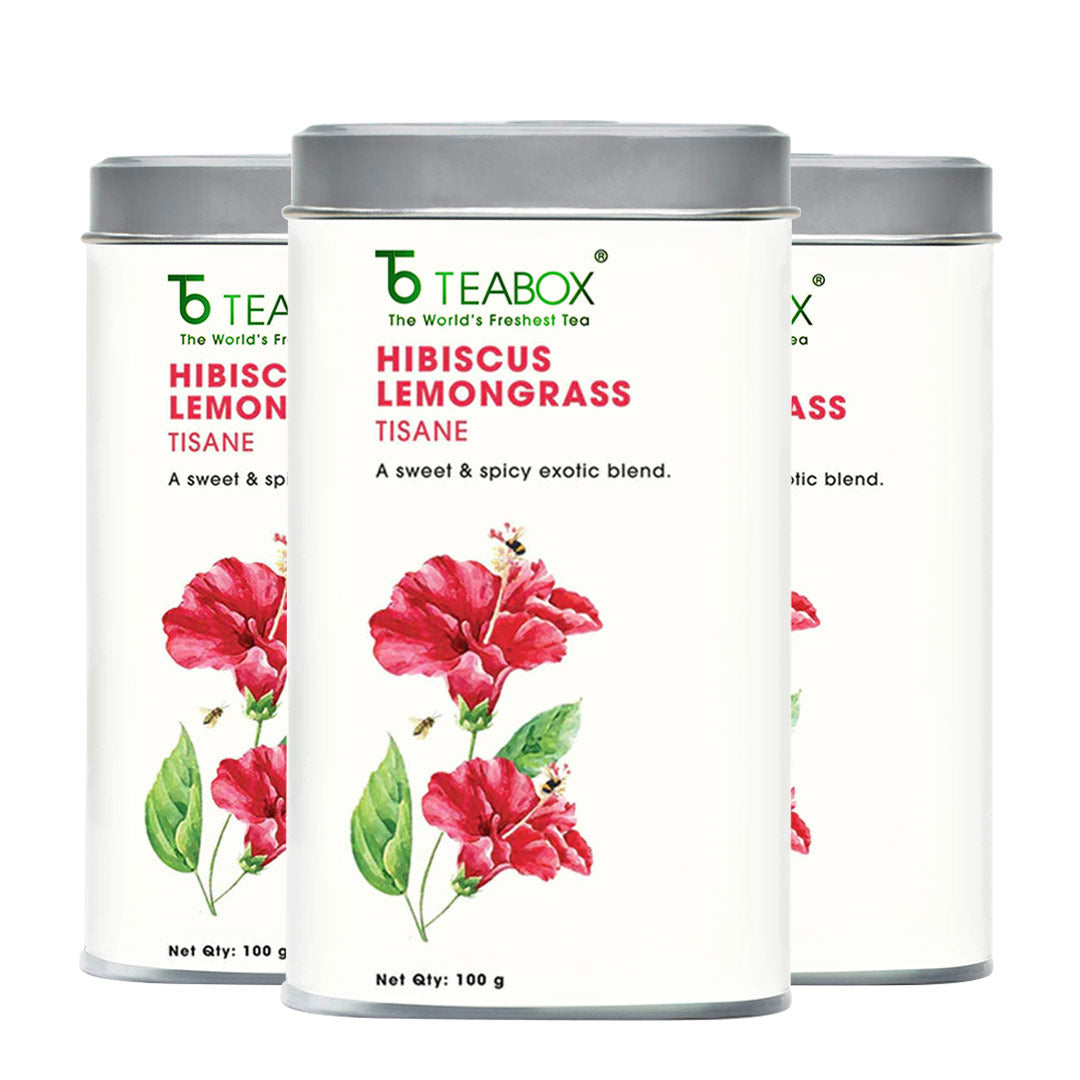The photograph depicts three identical tins of tea from the brand Tea Box, known as the world's freshest tea. Each tin is primarily white with a small silver lid at the top and a silver rim at the bottom. The tins are square-like in shape with curved edges. 

At the top of the tins, the brand name 'Tea Box' is printed in green, followed by the slogan 'the world's freshest tea.' Below this, the flavor 'HIBISCUS LEMONGRASS TISANE' is prominently displayed in all caps and in reddish-pink letters. Beneath the flavor name, the description 'A Sweet and Spicy Exotic Blend' is provided in smaller black text. An illustration of a hibiscus flower with two pink and red blooms and green leaves adorns the front of the tin. At the bottom, the net weight is listed as 100 grams in black font.

The arrangement shows one tin in full view at the front, with the left side of one tin and the right side of another tin partially visible behind it. The background of the tins is white, making the vibrant colors of the text and flower illustration stand out.